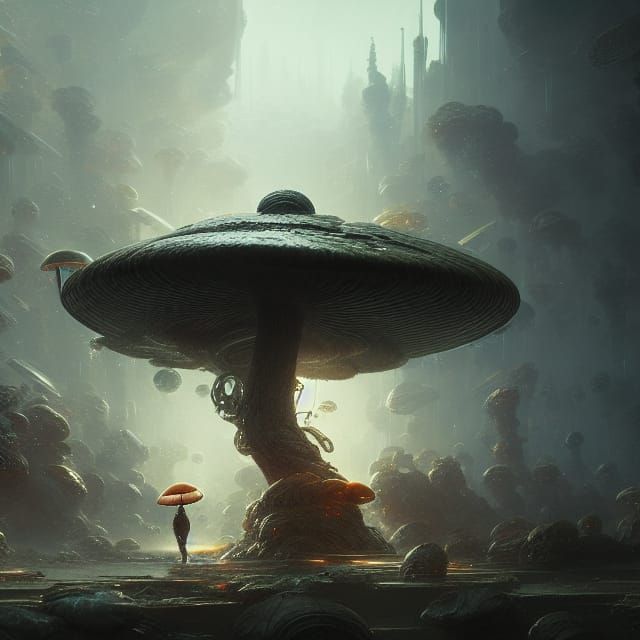In this digitally rendered, fantasy-inspired illustration, the scene is dominated by a colossal mushroom that stands at the center. The large mushroom, resembling the height and grandeur of a very large tree, has a massive stalk that supports a wide cap, which forms a canopy-like structure. The mushroom’s color ranges from gray to brown, with light hitting and reflecting off its top, creating a luminous effect. Below this giant mushroom, there is a smaller one with a vivid red cap.

The background is filled with a plethora of mushroom-like shapes, creating an almost mystical ambiance. On either side of the image, there seem to be cliffs or walls densely covered with mushrooms, adding to the surreal atmosphere. The floor of this scene appears to be uneven, populated by additional smaller mushrooms. Additionally, the light in the scene permeates from the top center, casting an ethereal glow that enhances the foggy, somewhat blurred edges of the image, particularly on the right side where vague, tower-like structures are visible but out of focus.

The illustration also features a silhouette of a figure in the foreground, possibly holding a red umbrella or another small mushroom. This figure, too, is bathed in the enigmatic light that shines from behind, accentuating the dreamlike quality of this imaginative, mushroom-filled landscape.